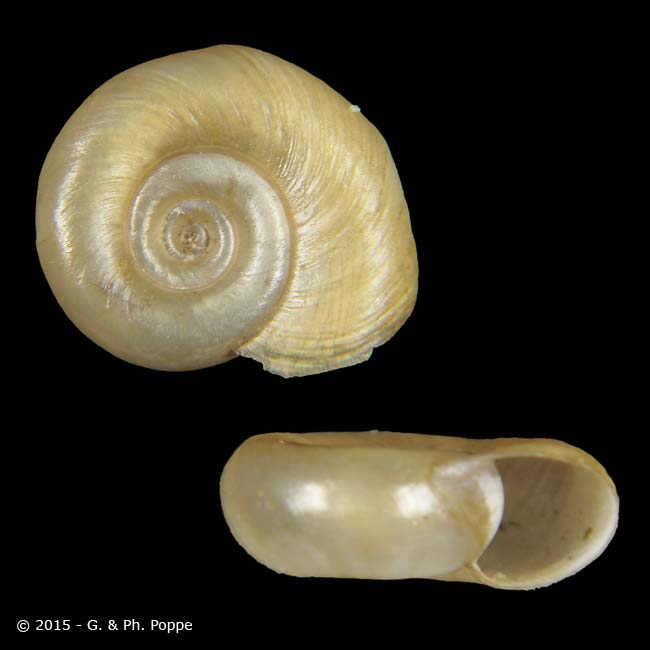This photograph showcases an empty snail shell, artistically depicted from two different angles against a stark black background. The shell, with its golden-brown, beige, and yellowish tones, spirals elegantly like a circular staircase, exhibiting a polished sheen that suggests professional varnishing. The top left quadrant displays a profile view of the shell, highlighting its intricate swirls, while the bottom right quadrant presents a view of its open, empty bottom edge. In the bottom left corner of the square image, the white text denotes a copyright mark: "2015 GMPH Puppy." The monochromatic backdrop and soft, even lighting give the photograph a refined, professional studio quality, enhancing the shell's natural beauty and detailed structure.